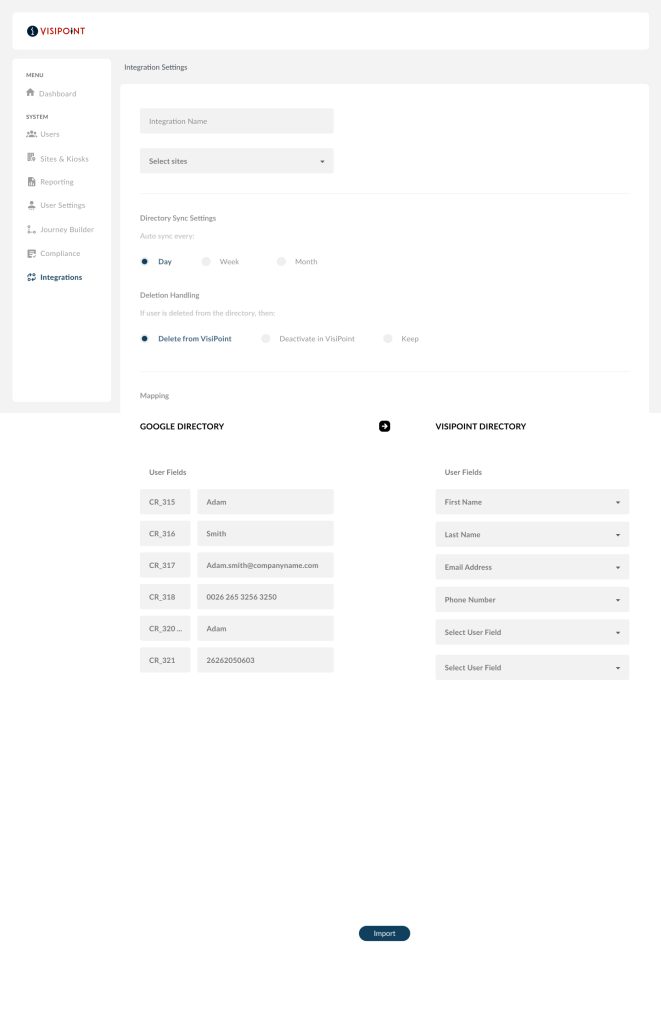The screenshot displays a structured layout with multiple sections and elements. At the top, there is a light gray square encompassing a horizontal white rectangle. Centered within this rectangle on the left side is a logo and a company name, which appear in red and blue.

Beneath the company name, a vertical white rectangle extends down the left side of the screen, featuring an unreadable list of items topped by a title, with icons and their names aligned next to one another.

To the right of this vertical white rectangle, a thin light gray horizontal strip runs across the screen. Below this strip, another large white rectangle fills the remaining area down to the bottom of the initial top square. In the upper left corner of this larger white rectangle are two stacked horizontal light gray rectangles, each containing black text.

A very thin blue line separates these gray rectangles from the section below. This lower section begins with a bold black title, followed by a line of black text and three horizontally-aligned choices, each accompanied by a selection button. A second identical set of choices lies directly below the first.

At the bottom of the screen, two boldly labeled columns appear. Under these headings, each column contains a list divided into two rectangles: a smaller gray rectangle and a longer horizontal rectangle next to it.